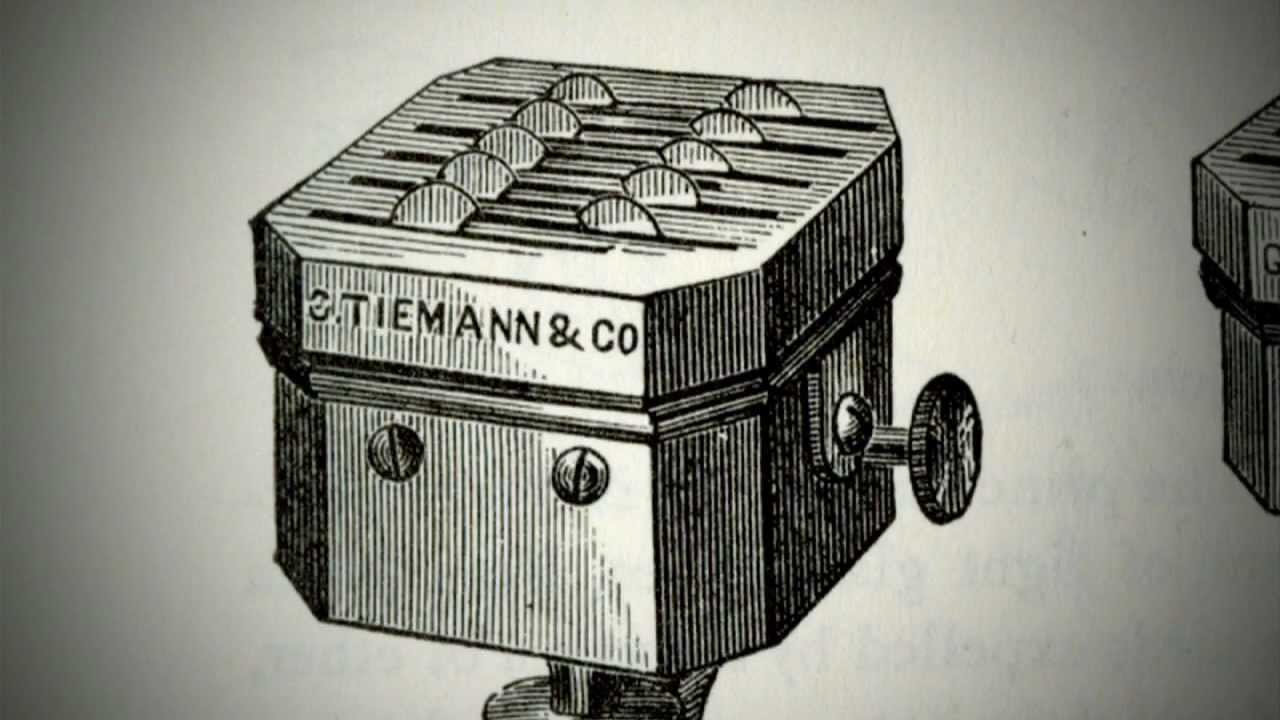This black and white hand-drawn image features a detailed mechanical box with a square, cube-like structure and beveled edges. The box has a lid, possibly indicating that it can be opened or separated. Inscribed on the front panel is the text "C.T.M. Tie Men and CO," with two screws visible below this text. The right side of the machine includes a round knob or crank. The top of the box displays multiple vertical slits, from which some round, wheel-like structures partially emerge. Surrounding the edges of the picture is a gray background, with a portion of another machine faintly visible on the right side. The black ink lines and arches contribute to the texture and depth of the drawing, enhancing the intricate mechanical and geometrical details.